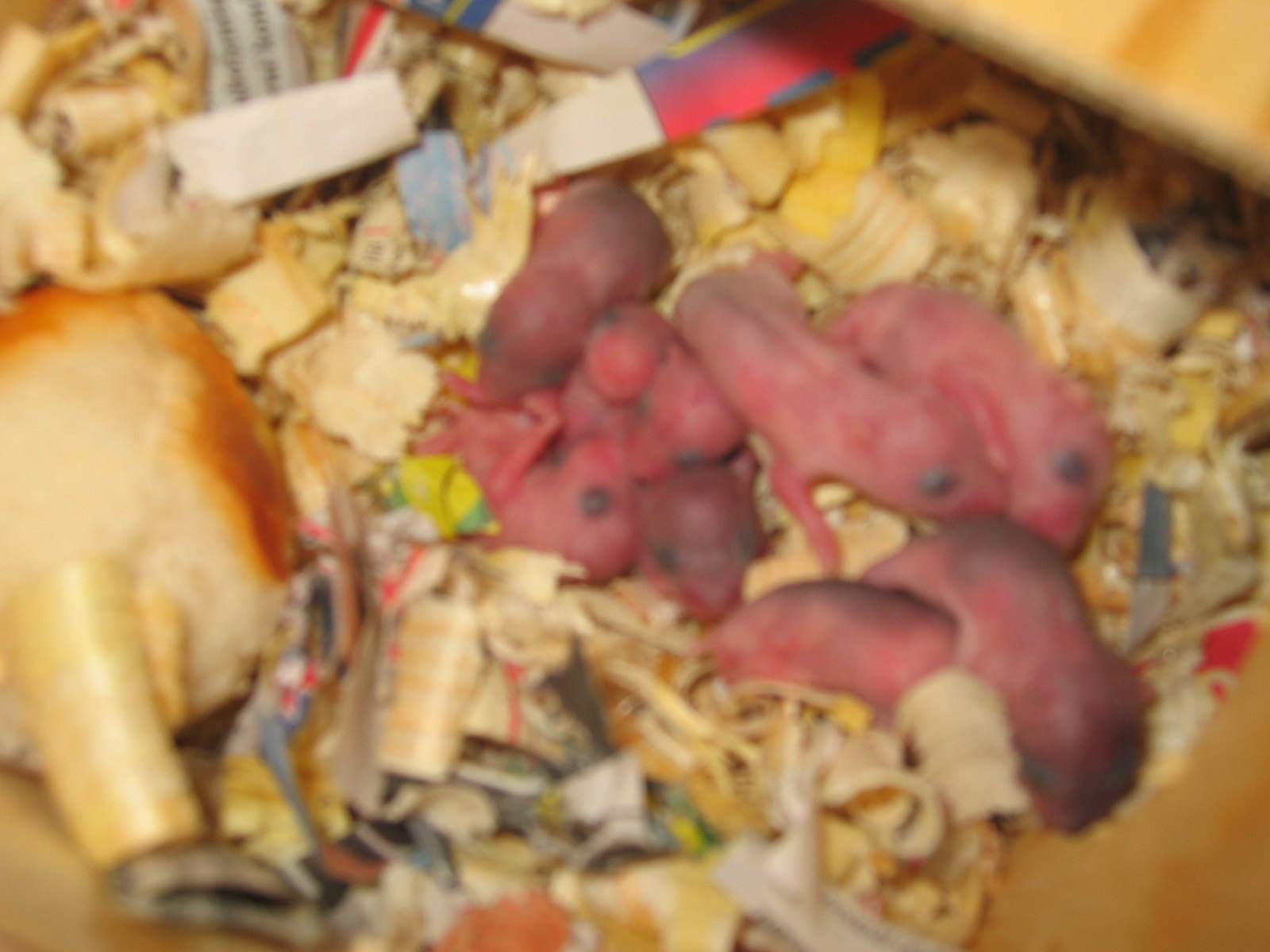This color photograph, although slightly blurred, captures nine newborn baby animals—possibly rats, mice, hamsters, or gerbils—huddled together in an enclosure. The infants are pink and hairless with undeveloped, closed eyes appearing as small dark dots on their faces. They rest on a bed of wood shavings mixed with variously colored paper fragments in shades of pink, white, and blue. To the left side of the image, there is an ambiguous object resembling a roll or possibly a piece of bread, although its exact nature is unclear and no mother animal is visible in the scene. The overall impression is of newly born, vulnerable creatures in a prepared habitat.